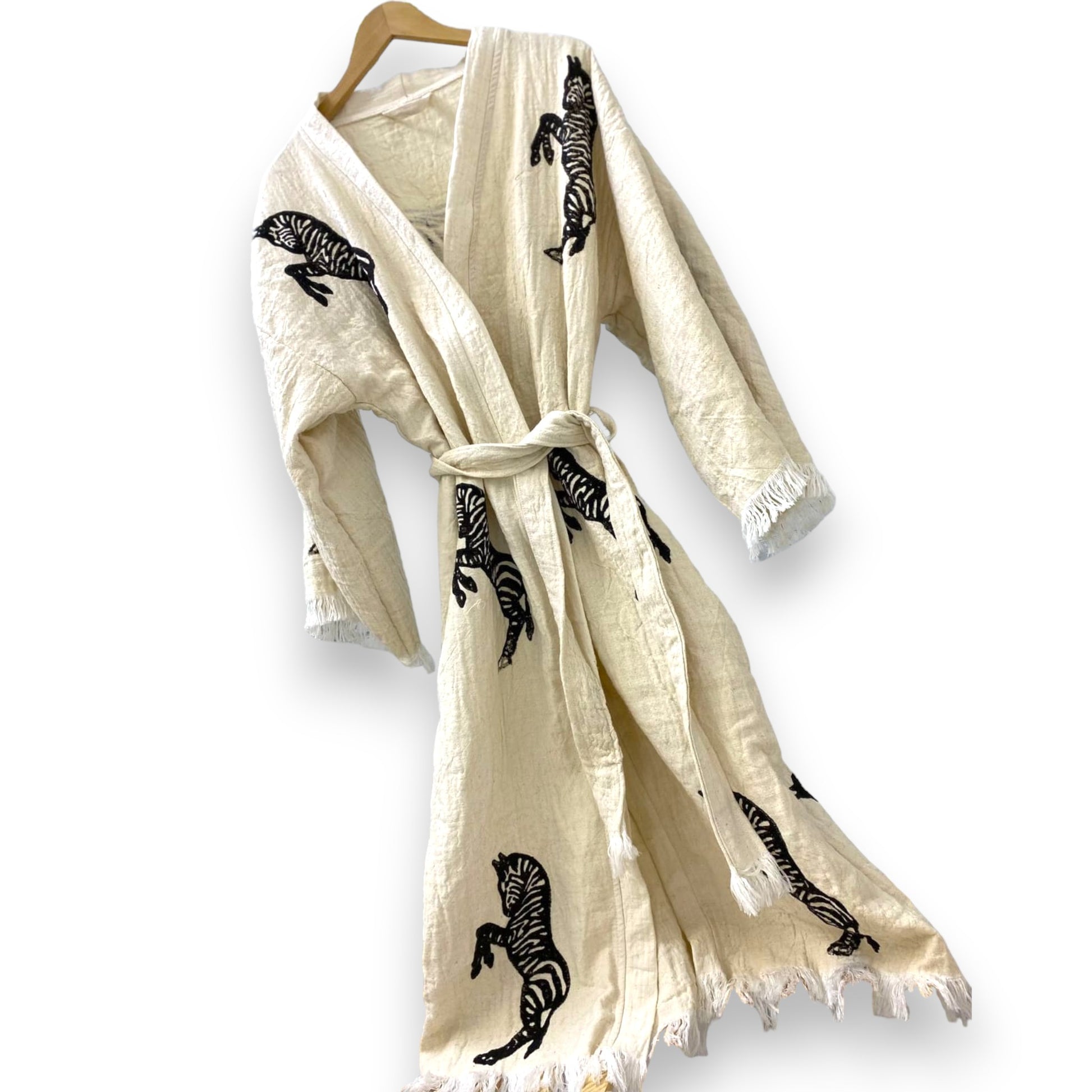This image showcases a beautifully detailed bathrobe suspended on a wooden hanger against a plain white background. The robe is a lush, cream-colored piece of merchandise that exudes elegance and luxury. It appears thick and soft, made from a textured, rugged linen-like fabric. The robe's defining feature is its intricate hand-knotted tassels that adorn the cuffs of its sleeves, the ends of the waist tie, and the hemline, adding a sophisticated touch much like the fringe on a Persian rug. Additionally, the robe is embellished with approximately six minimalist, black-embroidered zebras that stand about eight inches long, scattered across the front from the shoulders down to where the knees would be, spaced with ample white space in between them for a subtle decorative element. The overall presentation of the robe, captured in this product photo, highlights its flowing silhouette shaped by the tied waist, inviting viewers to imagine how it would drape elegantly on a person.